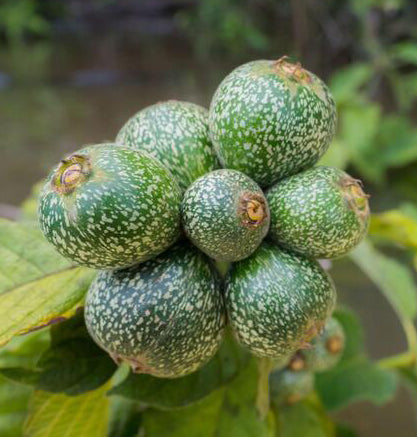The image displays a close-up of a cluster of round, greenish-white pods, possibly immature berries or fruits, nestled among green leaves. The pods, which resemble moldy grapes or unripe blueberries, exhibit a speckled pattern with white sprinkled across their green base, giving them an almost moldy appearance. Each pod has small brown sections at the top, likely indicative of areas where seeds may sprout. The background is entirely blurred, emphasizing the vibrant, detailed cluster of approximately eight pods and leaves in the foreground. The image's overall tone is very green, capturing an intimate view of these peculiar, early-stage fruits or vegetables.